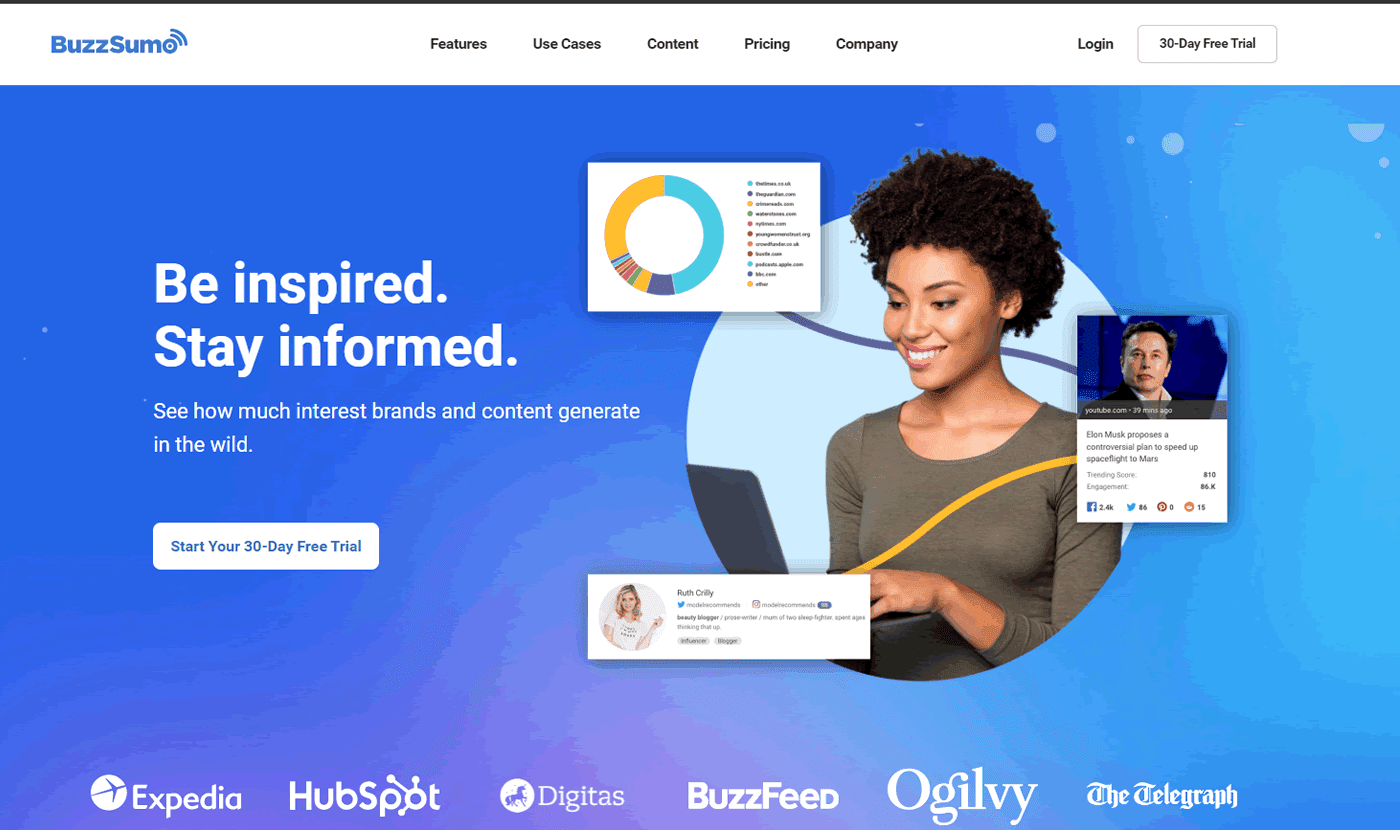Here's a cleaned-up and detailed caption for the described image:

---

This is a screenshot of the BuzzSumo homepage. At the top of the page, a white banner header prominently displays the BuzzSumo logo in blue text. To the right of the logo, in black text, are tabs for navigation: "Features," "Use Cases," "Content," "Pricing," "Company," "Login," and "30-Day Free Trial."

The main content area features a space-themed design with a blue background. In large white text, the headline reads "Be Inspired." Below this, additional text states "Stay Informed" and follows with "See how much interest brands and content generate in a wild." Positioned underneath this text is a prominent call-to-action button labeled "Start your 30-day free trial."

In the center of this blue background, there is an image of an African-American woman, smiling and looking to her left at a laptop. Surrounding her are various floating text boxes that provide context to her work environment. One text box contains an image of Elon Musk along with the text "Elon Musk proposed controversial plans to speed up space flight to Mars." Another box includes a tweet from someone named Ruth. Additionally, a circle bar graph is visible, though the text accompanying it is unreadable.

At the bottom of the screenshot, logos of well-known digital brands are displayed, including Expedia, HubSpot, Digitas, BuzzFeed, Ogilvy, and The Telegraph, emphasizing the platform's credibility and user base.

---